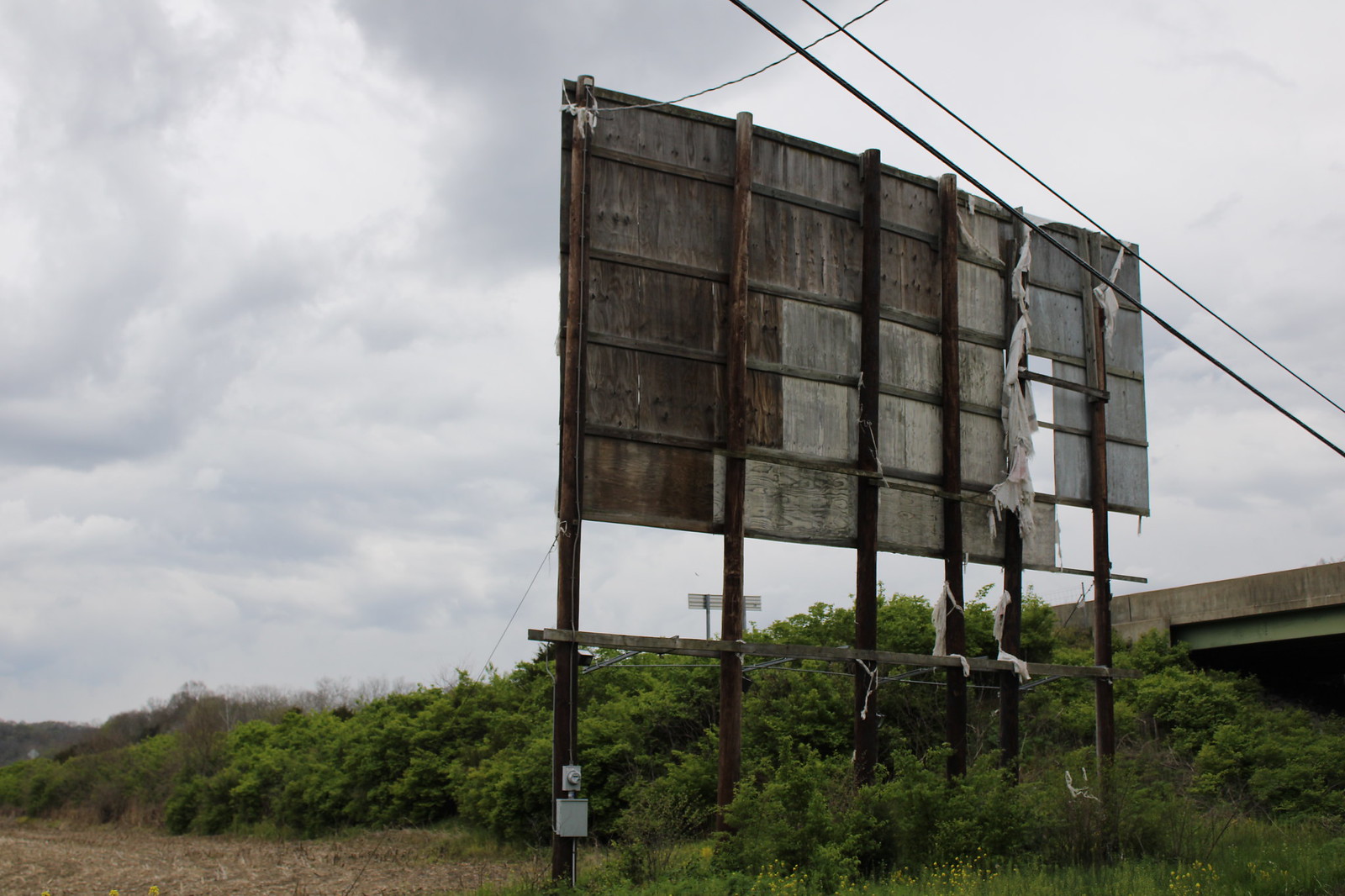The image captures the backside of a weathered, abandoned billboard, devoid of any advertisements or text. The structure is constructed from six unevenly spaced, vertically aligned wooden poles, supporting a rectangular piece of wood at the top. Noticeably, the right side of the billboard is missing several wooden planks, contributing to its dilapidated appearance. Hanging from the second pole on the right are tattered sheets of white cloth, fluttering in the breeze. An electrical box and meter are affixed to the base of the leftmost pole.

The foreground is a lush tangle of green bushes and shrubs, contrasted by patches of dead grass in the lower left corner and vibrant green grass sprinkled with yellow flowers in the lower right. The background reveals a calm, blue sky dotted with clouds, signifying a clear daytime setting. On the right side, a street or bridge is visible, partially obscured by electrical wires stretching across the upper part of the image.